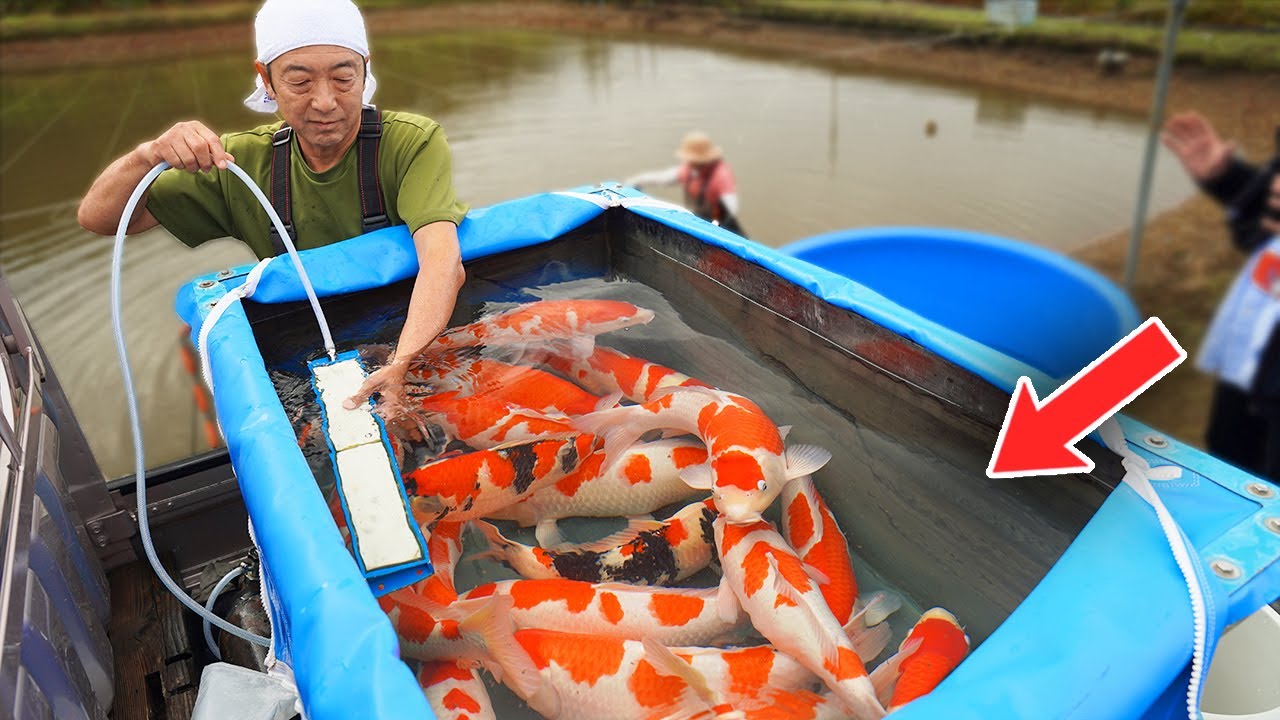A man, dressed in a green t-shirt and a white hat that extends down his back, stands in a boat that has a grey front and black sides, positioned on a green river. He is tending to a large makeshift blue tank filled with koi fish. These koi are notable for their long, white bodies adorned with bright orange and occasional black patches. The fish, which look to be a foot to a foot and a half long, and quite wide, are packed into the tank, which is either wooden or vinyl. The man is using a long rectangular white device connected to the tank by a narrow tube, possibly a filter or an air-providing mechanism to maintain oxygen levels, or perhaps measuring the water's temperature. Surrounding this busy scene, the background reveals a man-made pond with dirt and grass edges, a man’s hand, possibly another fisherman, and another blue tank that may contain more koi. A prominent red arrow points to the koi from the right center of the image.